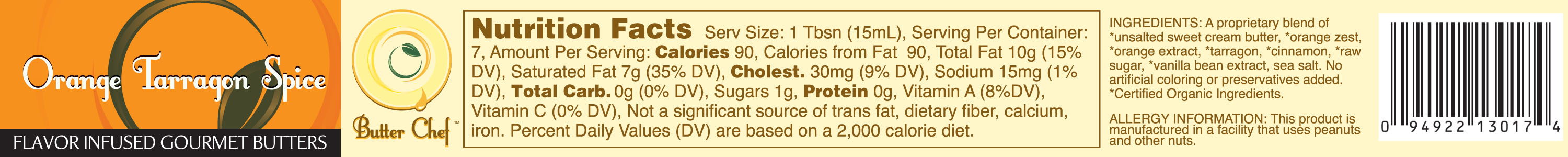The image displays a nutrition label for Orange Tarragon Spice Flavor Infused Gourmet Butters. The label prominently features an orange background with white text, and at the bottom, a black strip delineates the product's name. To the right of this design is the detailed nutrition information.

The label specifies the following nutritional values per serving (1 tablespoon):
- Servings per container: 7
- Calories: 90
- Total Fat: 10 grams
- Saturated Fat: 7 grams
- Cholesterol: 30 milligrams
- Sodium: 15 milligrams
- Total Carbohydrates: 0 grams
- Sugars: 1 gram
- Protein: 0 grams
- Vitamin A: 8% of Daily Value
- Vitamin C: 0% of Daily Value

The label also notes that the product is not a significant source of trans fat, dietary fiber, calcium, or iron. Percent Daily Values are calculated based on a 2,000 calorie diet.

Adjacent to the nutritional facts, the label lists the ingredients, although they are hard to discern due to the small print size. Below the ingredients section, there is an allergy information disclaimer stating that the product is manufactured in a facility that processes peanuts and other nuts.

Finally, a barcode is situated next to the ingredients and allergy information.